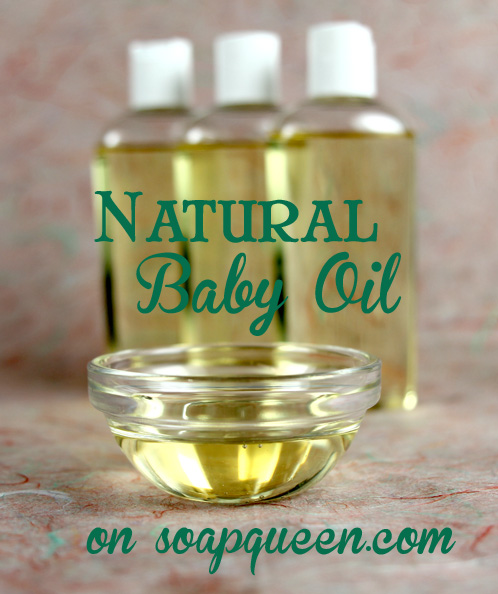This vertical rectangular image serves as an advertisement for baby oil, prominently marketed on SoapQueen.com. The focus of the image lies on three clear bottles, each filled with a yellow liquid and capped with white lids. These bottles, arranged in a row, prominently display the product name "Natural Baby Oil" in large, green cursive letters, with the word "natural" highlighted in a larger font. In the foreground, a small dish—approximately halfway filled with the same yellow liquid—accompanies the bottles. Beneath the dish, the text "on SoapQueen.com" is written in cursive green letters, suggesting the product's availability on the website. The entire setup is placed on what appears to be a granite or marble countertop, adding a touch of elegance to the scene. The cohesive use of green lettering in various fonts ties the image together, emphasizing the natural theme of the baby oil.